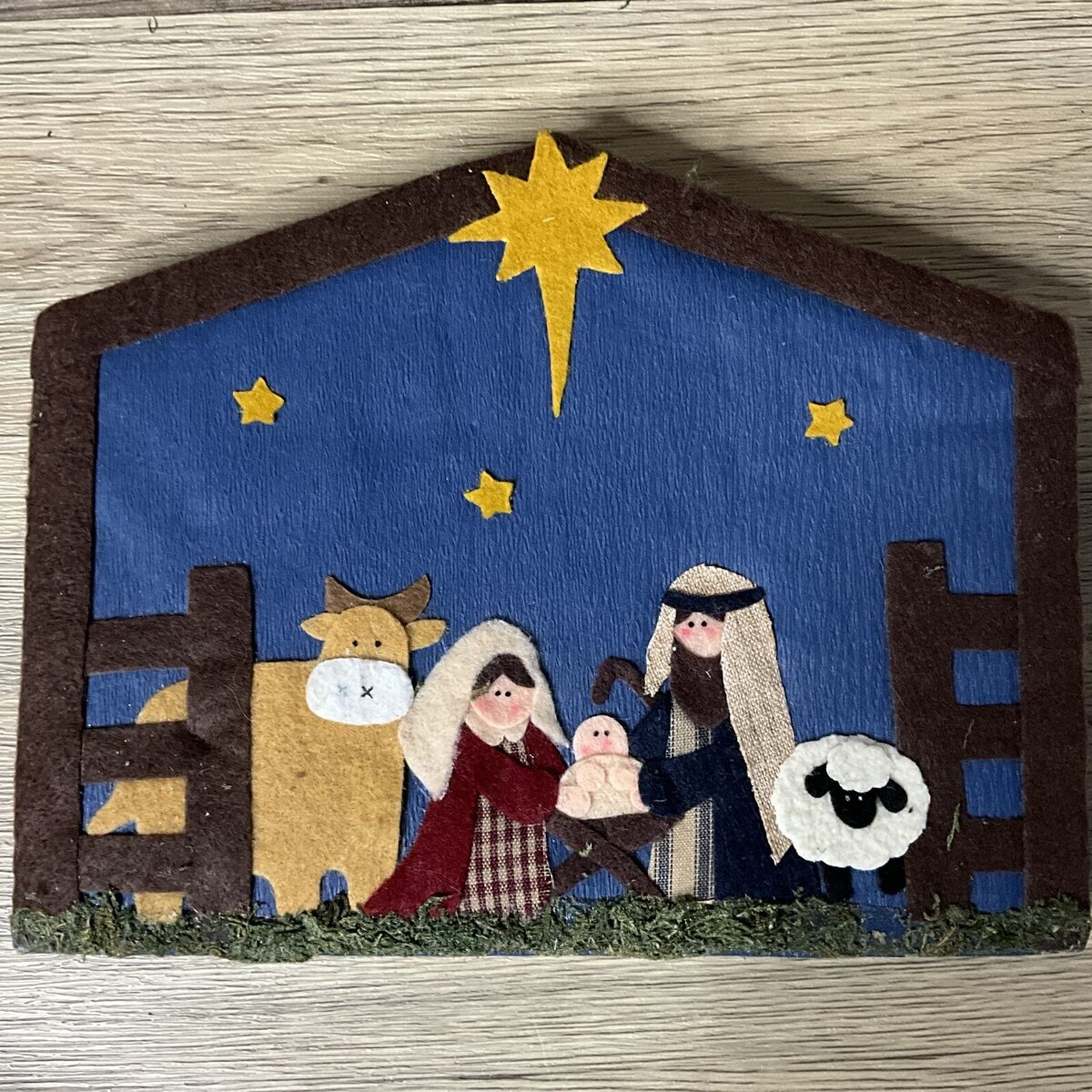This image depicts a handcrafted nativity scene, created with a folk-art style using felt and cloth cutouts. The scene is set within an A-frame manger structure, crafted from brown cloth, and framed by what appears to be bleached wood. The background is a dark blue sky adorned with several golden, textured stars, including one prominent star above the manger. At the center, the baby Jesus is swaddled in white cloth, with only his head visible. Mary is dressed in a burgundy overcoat and a red-and-white checkered dress, with her head covered. Joseph, often mistakenly called Joshua, has a long brown beard, a headdress, and a blue shawl. Surrounding them are animals, including a cow with horns and a sheep, both made from felt. The scene is further detailed with green felt grass below the figures, adding texture to the composition. The entire depiction rests on a wooden counter, completing the rustic, handcrafted aesthetic.